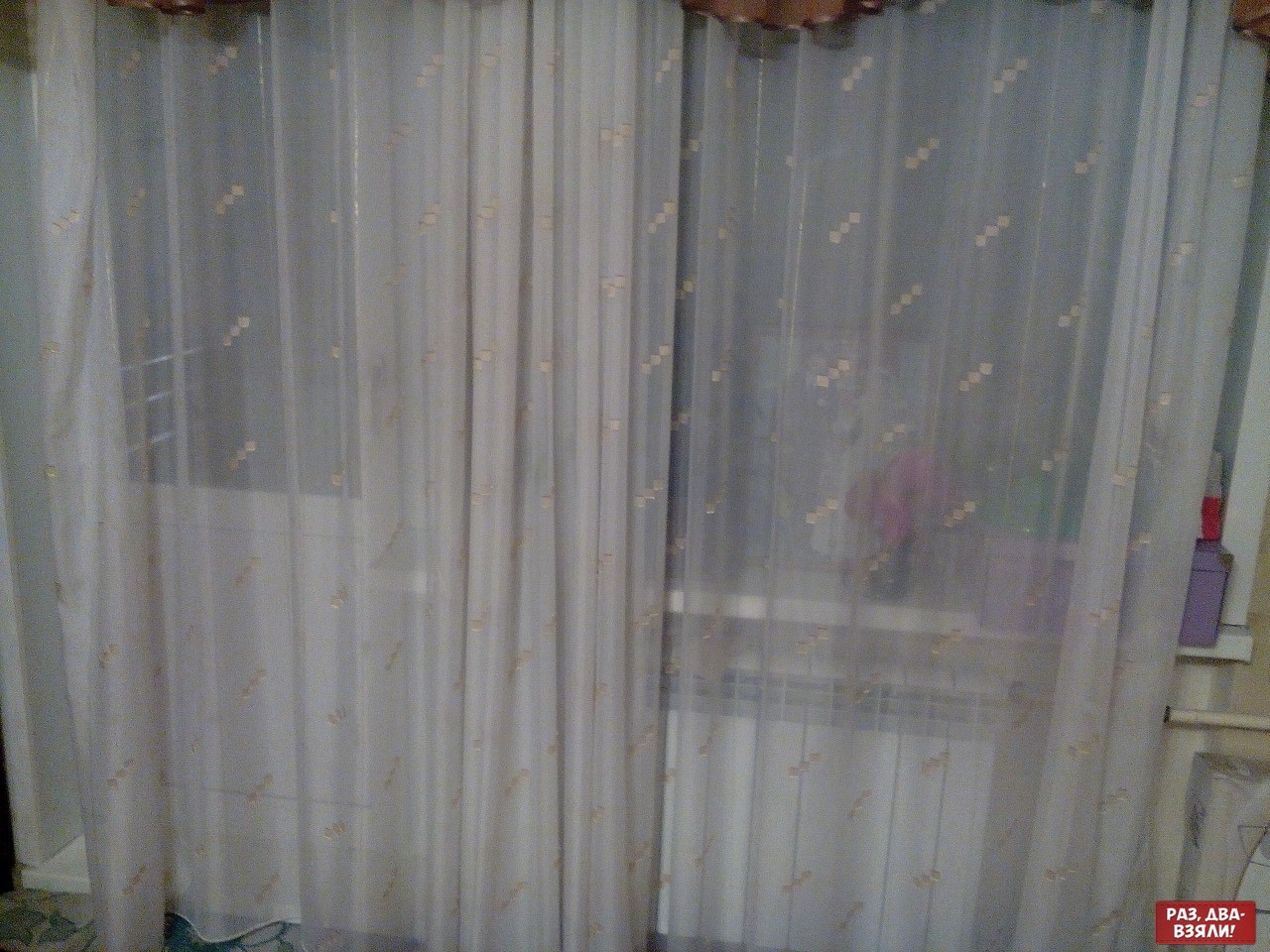This photograph, taken inside a house, focuses primarily on a large, off-white thin, silky curtain with a repeating design of golden, pixelated blocks arranged horizontally. The curtain, which has visible ruffles and wrinkles, hangs from the top to nearly the bottom of the image, close to the floor. Behind this translucent curtain, a window is partially visible, framed by a white wall. A cluttered windowsill can be seen, featuring a prominent purple box, a small vase of flowers, and several picture frames, with indications of a photograph, possibly a wedding day image. On the right side of the image, there's a red box with white text in another language, stating "PA3ABABRAN!" with an exclamation mark. Additionally, to the left, there's a glimpse of what appears to be a screen door, indicating a possible porch area.